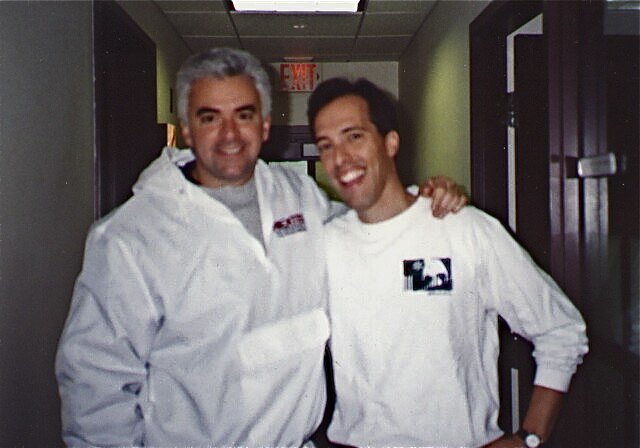The photograph features two Caucasian men standing in an indoor hallway that resembles an office environment. The hallway features a tiled ceiling, with visible fluorescent lighting and white or off-white walls. In the background, there is a prominently lit exit sign with red letters positioned above a brown door. The man on the left, who is noticeably taller and with grayish-white, short-cropped hair, is smiling and wearing a white pullover hoodie with an emblem that isn't clearly visible. He has his arm around the slightly shorter man on the right. This shorter man has dark brown hair, brown eyes, and is adorned in a white long-sleeved t-shirt, also smiling warmly. The photo, seemingly dated and possibly from the 90s, appears to be a scanned or reprinted copy from a physical medium such as a magazine or newspaper. Both men stand close to each other, suggesting a friendly or familiar bond, evident by their relaxed and affectionate posture.